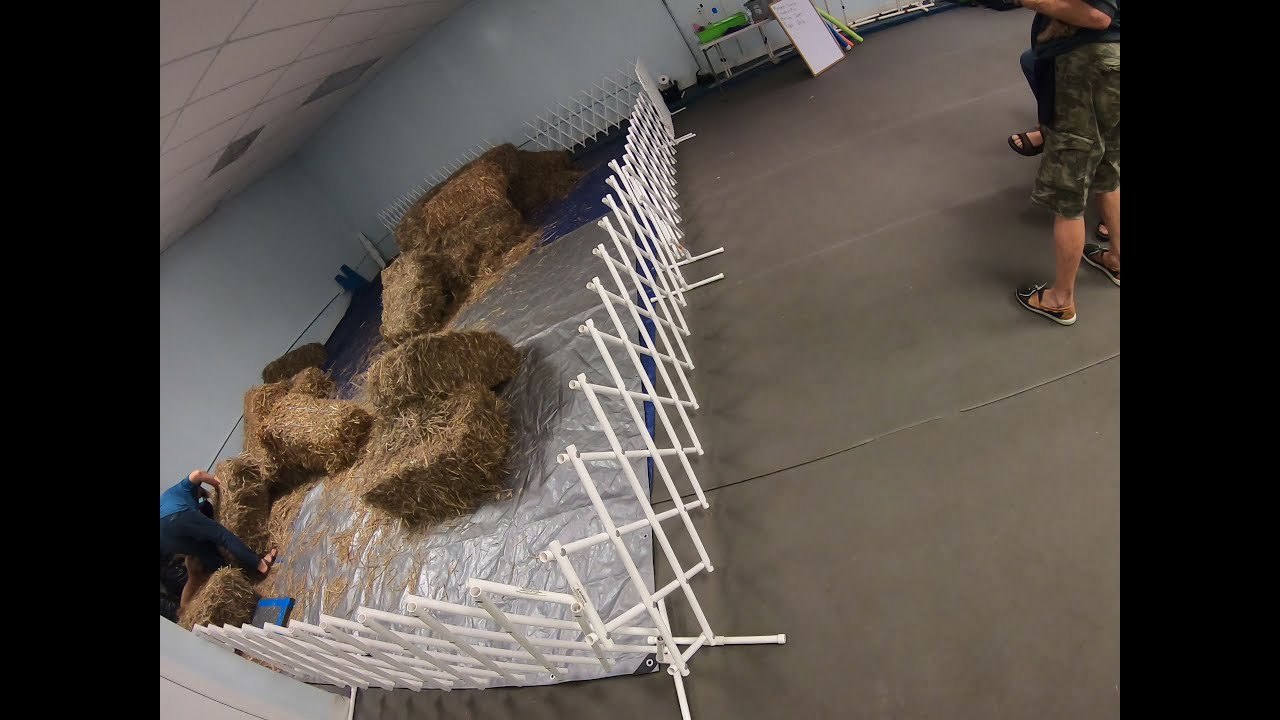The image depicts an indoor scene featuring several hay bales scattered haphazardly on a shiny gray tarp, enclosed within a white, temporary, crisscross diamond-patterned fence. A man in a bright blue shirt and dark blue pants is bending over the hay bales, suggesting he might be organizing them. To the right side of the photo, the lower halves of two other men are visible, both wearing sandals, with one distinguishable by his dark green shorts. In the background, the scene includes a white chalkboard and colorful swimming pool noodles. The floor appears to be a hard concrete surface, and the overall setting might be a farm storage area or some indoor animal facility, though no animals are visible in this image.